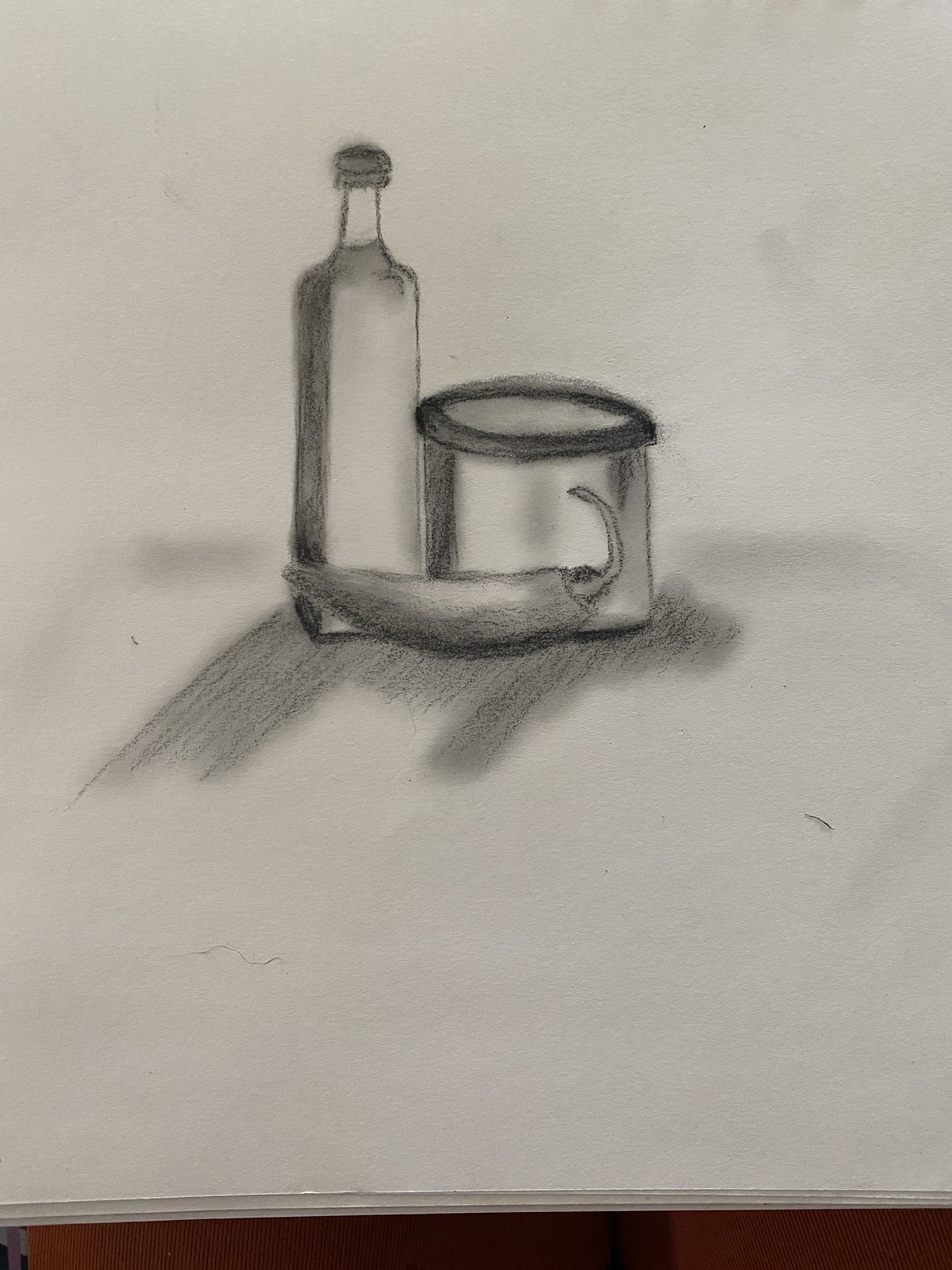A detailed pencil drawing, rendered in varying shades of gray and black, sits on a slightly gray piece of paper. This paper is placed atop two additional sheets of white paper, all positioned on a brown wooden table. The central focus of the drawing is an olive oil bottle, appearing full and capped, without a label. Next to the bottle, there is a round metallic container—possibly a measuring cup or similar vessel—lacking a handle. In front of these objects lies a whole, uncut chili pepper. Each item in the composition casts a distinctive shadow, enhancing the depth and realism of the artwork.